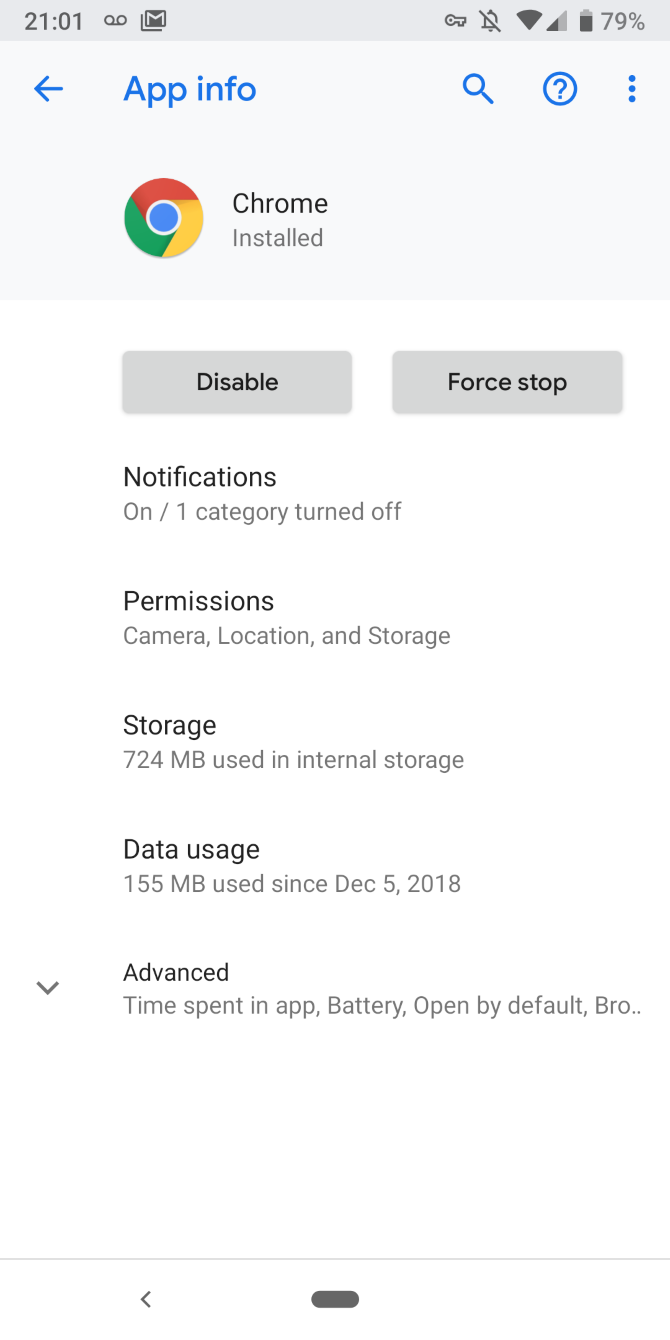**Detailed Description of a Cell Phone Screen Screenshot**

At the top of the screenshot is a medium gray border running horizontally, where the top left corner displays the time "21:01." In the top right corner, a set of icons is visible, including the battery icon indicating 79% charge and the cellular connection icon.

Below this gray border is a lighter gray banner featuring a left-pointing arrow next to the text "App Info." Beneath this, there is the Google logo accompanied by the words "Chrome" and "Installed."

The background of the rest of the screen is white. Two buttons with medium gray backgrounds are positioned side by side. The button on the left has centered black text that reads "Disable," while the button on the right also has centered black text, reading "Force Stop."

Following these buttons, there are five headings in bold black text:

1. **Notifications:** Displays "On / 1 Category Turned Off."
2. **Permissions:** Lists "Camera, Location, and Storage."
3. **Storage:** States "724 MB used in Internal Storage."
4. **Data Usage:** Indicates "155 MB used since December 5, 2018."
5. **Advanced:** Followed by "Time Spent in App, Battery, Open by Default, Bro..." with the text trailing off.

This detailed description captures all the elements visible in the screenshot, providing a clear and thorough overview of what is displayed on the cell phone screen.